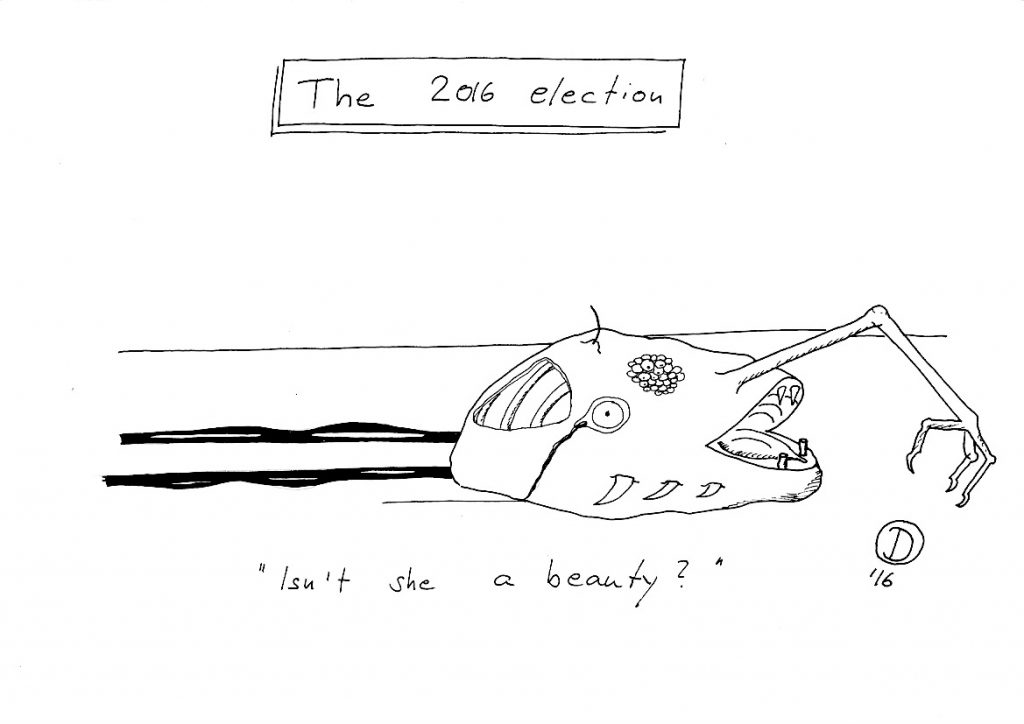This black and white pen-drawn political cartoon depicts a hideous, grotesque beast personifying the 2016 election. At the top, a thin, black rectangular banner reads "the 2016 election." Below, a monstrous skull leers, dragging itself forward with a single, three-fingered arm, leaving a dark trail in its wake. This malformed creature has an eyeball, an open mouth with fangs, exposed ribs, and scales, as well as spikes protruding from its distorted head. The back of its skull is partially missing, revealing more internal horrors. Overlying grotesque details such as a patch of fungus or blistery circles add to its repulsiveness. Below this unsettling image is the sarcastic caption, "Isn't she a beauty?" In the bottom right corner, the illustrator's signature is marked with a capital D in a circle and the notation "1/6."